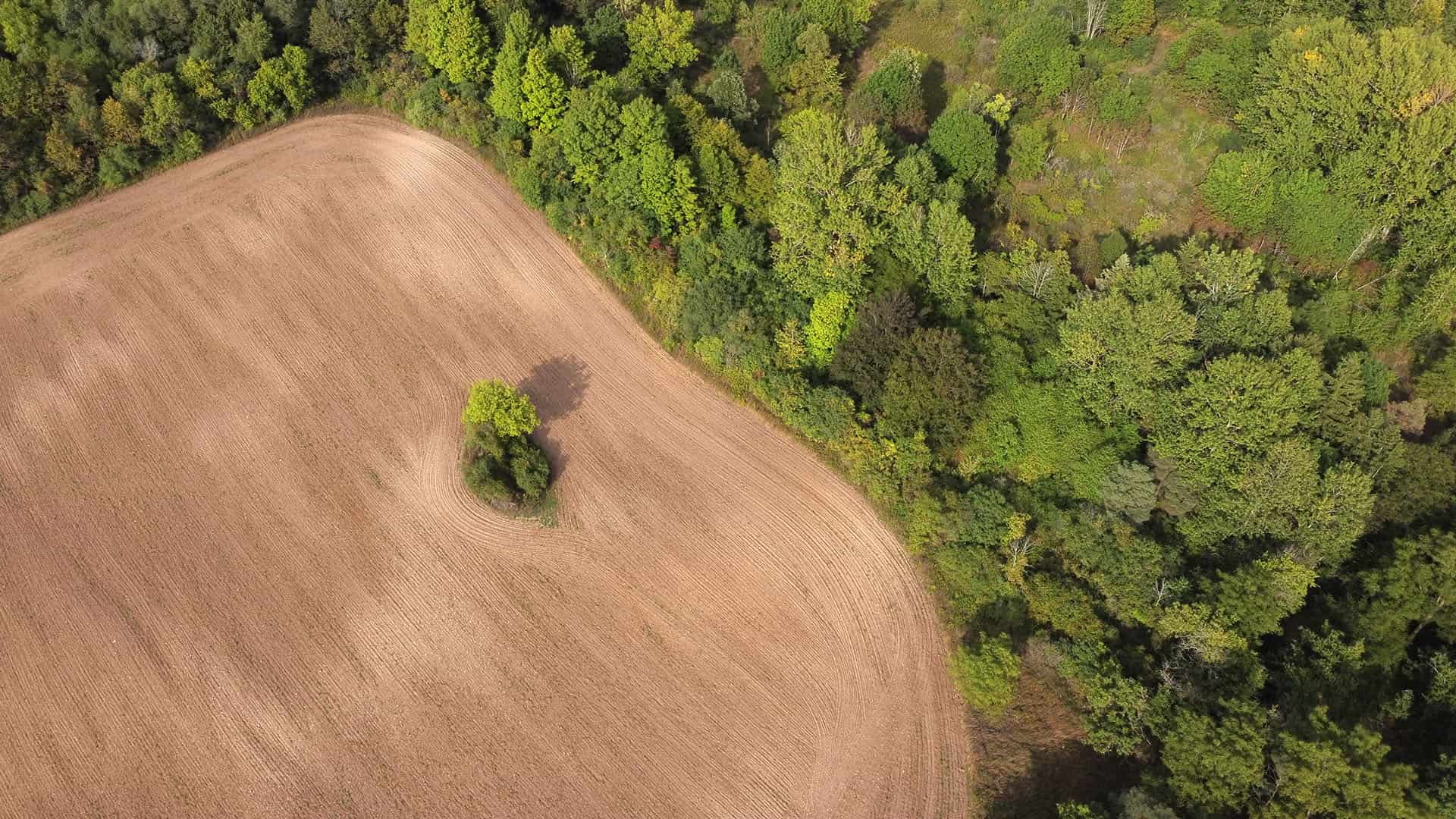This aerial photograph, taken from a high vantage point like a drone or airplane, depicts a vibrant outdoor nature setting. Dominating the left half of the image is an expansive field of raw, well-manicured soil. Nestled within this expanse are two to three trees, presenting a mix of light and dark green hues. The surrounding perimeter of the field is densely fringed with diverse stands of trees, exhibiting variations in height and leaf color from bright lime to deep emerald and including both deciduous and coniferous types. In the top right corner, a mixture of light and dark green trees is visible, enhancing the diversity of the forested border. The bottom right corner highlights a patch of black soil interspersed with trees. The scene, bathed in bright daylight, suggests clarity and warmth, emphasizing the contrast between the cultivated field and the wild, untouched forest.